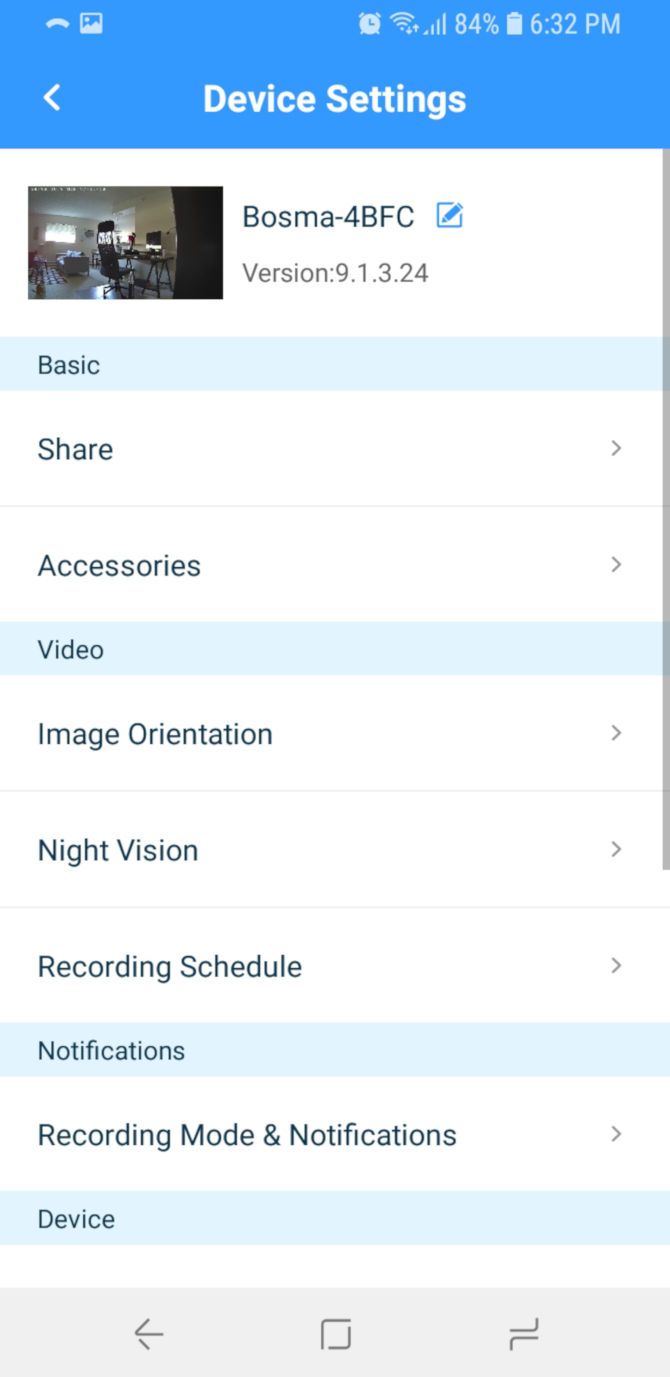This is a detailed screenshot from a mobile phone, displaying various device settings. The top section features a light purple header, showing the time at 6:32 PM, a fully charged battery, full Wi-Fi signal, strong mobile signal, and an alarm clock icon. Below this, in white font, "Device Settings" is displayed with a left-pointing arrow to its left.

Directly underneath, a white rectangle contains a small image depicting the interior of a home. This image is followed by the text "Bosma-4BFC version 9.1.3.24" in black font, accompanied by a pencil icon indicating the option to rename the device. 

The interface below consists of multiple bars: 
- A blue bar labeled "Basic"
- A white bar labeled "Share"
- A white bar labeled "Accessories"
- Another blue bar labeled "Video"
- A white bar labeled "Image Orientation"
- One more white bar labeled "Night Vision"
- A white bar labeled "Recording Schedule"
- Finally, a blue bar labeled "Notifications"

Each section provides specific controls and information related to the device's settings and functionalities.